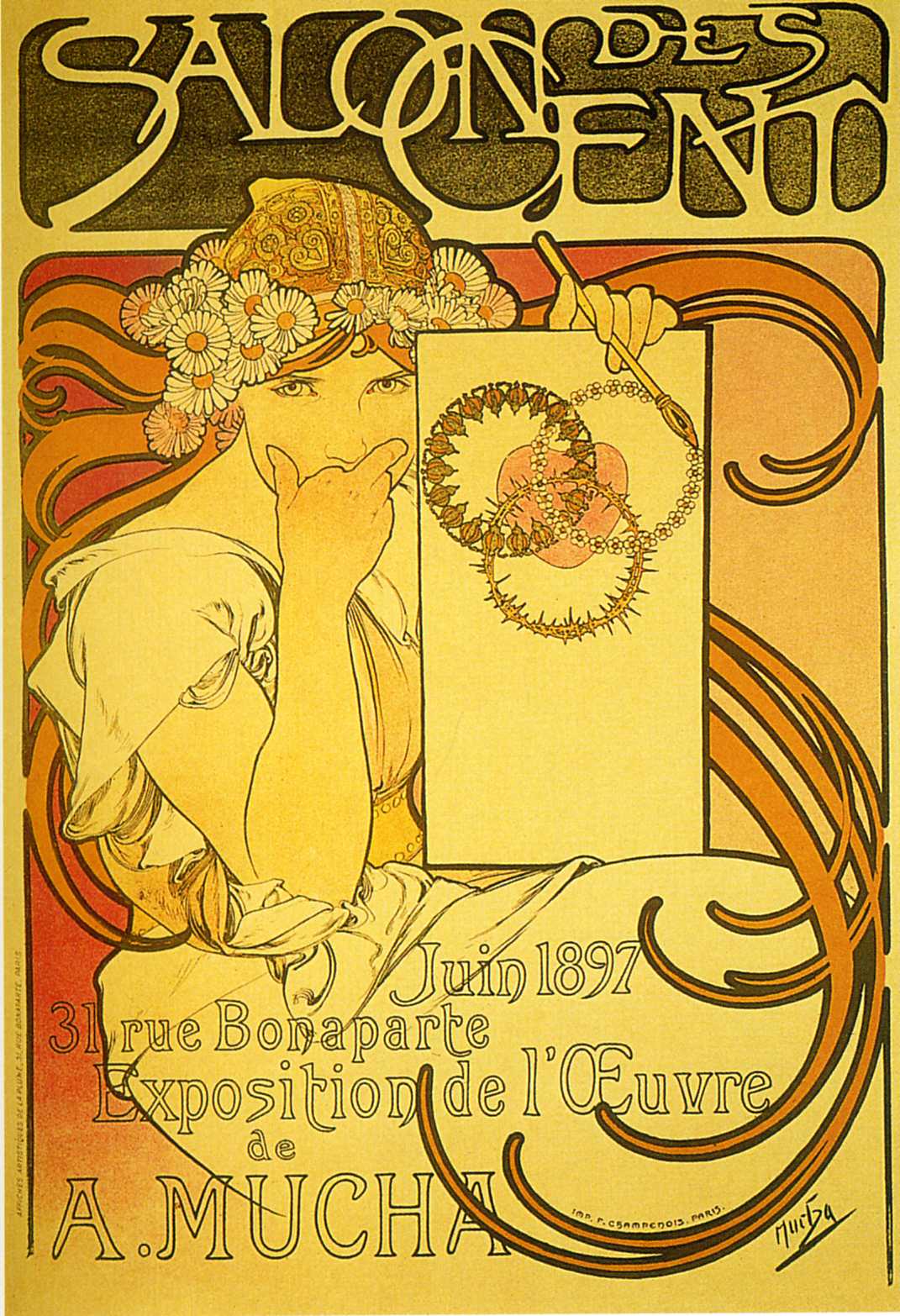This detailed drawing, designed to be made into a print, depicts a vintage-style poster for the "Salon des CENT" exposition. The setting is indoors, under a predominantly yellow background. At the top of the poster, the bold text reads "Salon des CENT." The central figure is a woman with a direct gaze, addressing the viewer. She adorns daisies in her blonde hair, and a short-sleeved white gown drapes elegantly on her form. She holds a paintbrush in her left hand, and with her right hand, she gestures upwards, covering her mouth.

In her left hand, the woman presents a drawing featuring three jagged, interconnected circles with a red heart in the center. Surrounding her figure are intricate orange swirls, adding a dynamic decorative touch. Inscribed at the bottom of the poster are the details: "Joanne, 1897, number 3, 31st Rue Bonaparte, Exposition de l'oeuvre d'Edouard Muchat." The artist's signature, "A. Mucha," is prominently displayed in the lower right-hand corner, indicating the creator's distinct handwriting style. This elaborate composition truly captures the essence of a historical art exposition, blending intricate details with bold text elements.